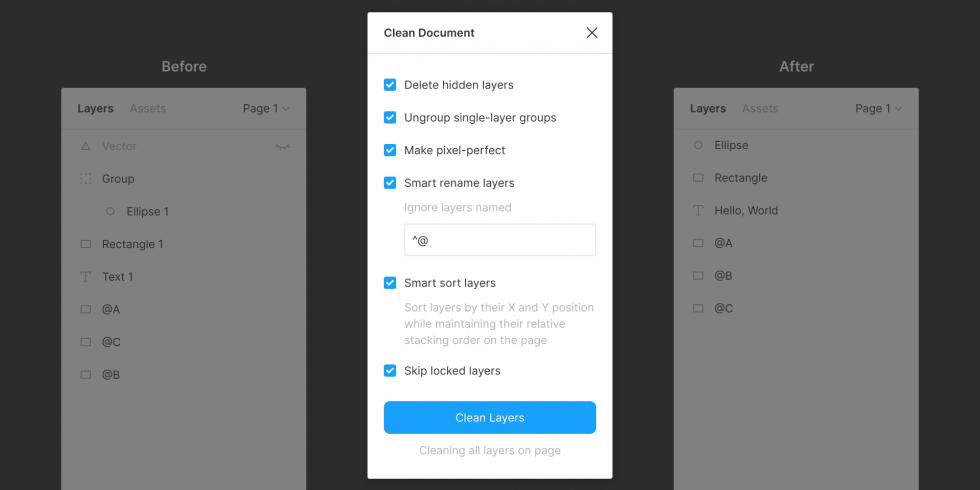The image is a screenshot taken from a smartphone or computer, showcasing a graphic design or layer management tool in use. The background of the image is a flat, solid black color, devoid of any texture or dimension.

On the left side of the image, there is a section labeled "Before" in white text on the black background. Below this, a white rectangular box displays the word "Layers" in black, followed by "Assets" in gray and "Page 1." Under these headings, there are a series of items listed vertically: "Vector," "Group," "Ellipse 1," "Rectangle 1," and "Text 1," each prefixed by a small, unchecked box.

In the center of the image, there's a prominent area labeled "Clean Document" accompanied by an "X" mark, possibly for closing the section. Below are several checkmarked options, each accompanied by descriptive text: "Delete hidden layers," "Ungroup single layer groups," "Make pixel perfect," "Smart rename layers," "Ignore layers named @," "Smart sort layers," and "Skip blocked layers." Each of these actions has a checkbox to the left, with all except "Ignore layers named @" being checked. At the bottom, there is a clickable button labeled "Clean Layers."

On the right side, the image mirrors the left, but under the section marked "After," we see a reorganized list consisting of "Ellipse," "Rectangle," and a text item labeled "T" with the content "Hello world." Below these items, the labels "@A," "@B," and "@C" are listed, similar to the "Before" section, with none of their boxes checked.

This image likely represents a comparative view of a document's layer structure before and after undergoing a cleaning process to organize and streamline its components.